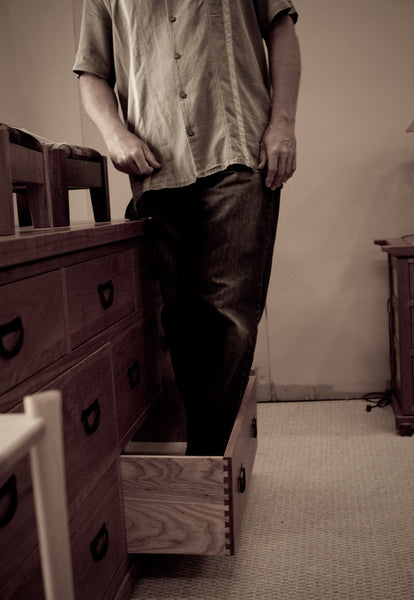In this sepia-toned image, a man is intriguingly positioned inside the bottom drawer of a wooden dresser, giving the photograph an old-fashioned feel. The dresser, constructed from a wooden material, stands prominently on the left side of the room, which features a carpeted floor and off-white walls. The man's head is not visible in the frame, but his body is clearly dressed in a short-sleeved button-down shirt with a stripe down the front, and a pair of pants, possibly jeans. His stance within the drawer, which is surprisingly open, shows his body slightly turned towards the camera as if demonstrating the sturdiness of the furniture. There is additional furniture partially visible in the background, adding to the domestic setting of the scene. The overall composition, though somewhat peculiar and monochromatic with a desaturated, brownish hue, evokes a sense of curiosity and timelessness.